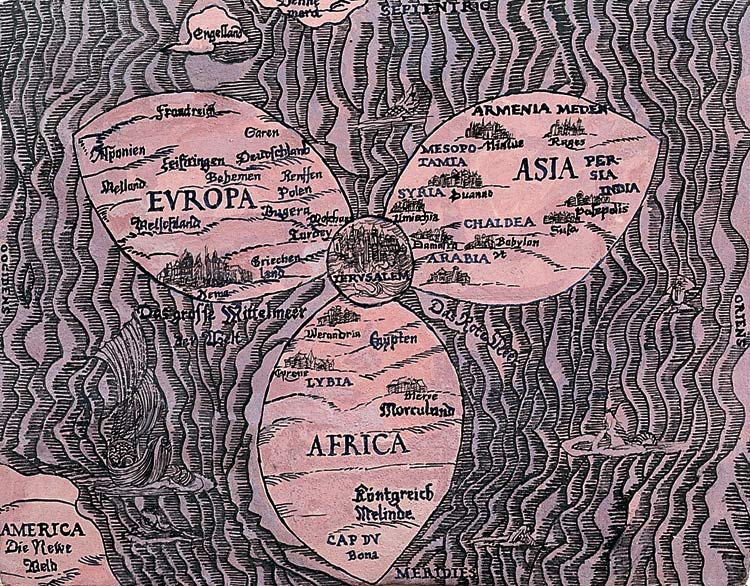This artwork, titled *Knowledge the World*, features a stylized, purple-toned map with a centrally placed, three-petaled flower design symbolizing a primitive depiction of the continents. The central round part of the flower is labeled "Jerusalem," connecting the three petals. The upper left petal, labeled "Europa" (Europe), includes names of numerous German towns. The upper right petal represents "Asia," listing regions such as Armenia, Chaldaea, Arabia, and Persia. The bottom petal signifies "Africa," with regions like Libya, Morocco, and Cap Bona marked on it. The map also includes distinguishable elements like a small island labeled "England" in the upper left-hand corner of the sea and a wavy-edged partial shape labeled "America" in the lower left-hand corner. The entire map is set against a pale pink background, shaded with gradient wavy black lines, which also contain additional tiny images and icons, like a swimmer in the bottom right and a flag mixed into the waves, creating an intricate and symbolic representation of the world revolving around Jerusalem.